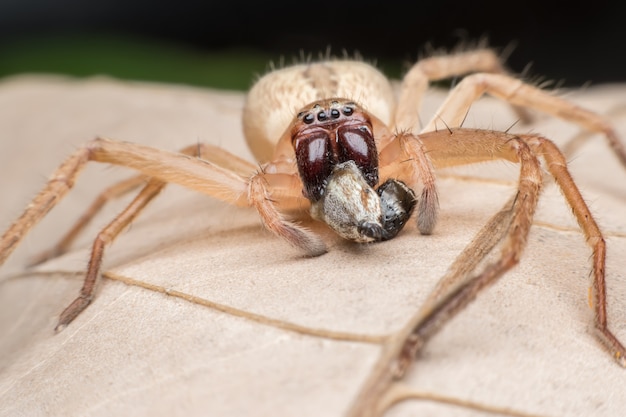The photograph showcases a detailed view of a spider resting on a tan brown leaf adorned with light-colored veins and dark stems. The spider, blending in perfectly with the leaf, is primarily tan with a smooth texture and various hairs and bristles covering its eight legs. Its abdomen is light brown with a large distinct brown spot, while the semi-transparent head features multiple round black eyes and pronounced dark brown mandibles gripping a white and black bug. The spider's coloration and body suggest it could be either a camel spider or a wolf spider, as it exhibits characteristics common to both. The rectangular image, with its blurred green background at the top, accentuates the spider's detailed features, making it a compelling and intricate close-up.